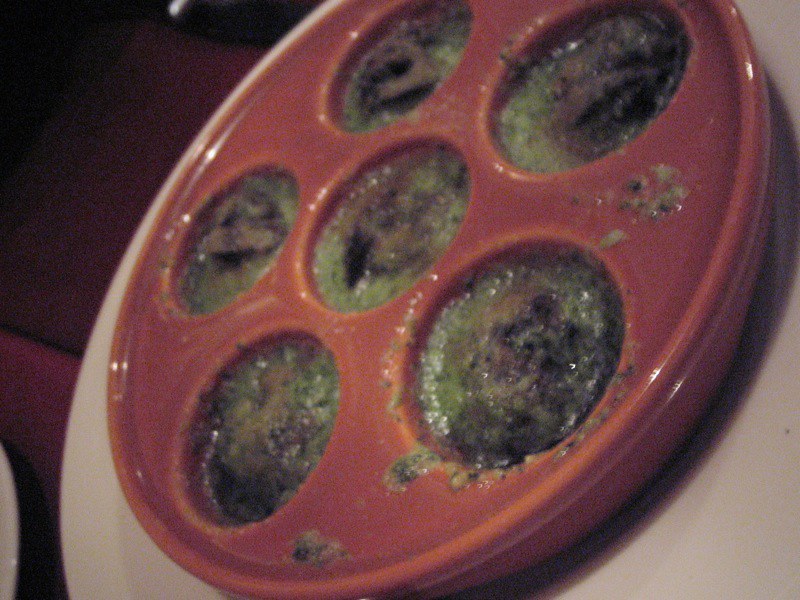In the center of the image is a reddish-brown, round tray resembling a film reel, with six circular dips arranged in a star pattern. These dips contain a greenish, brownish, and somewhat black mushy substance, likely some type of food like broccoli and mushrooms, with some fragments scattered on top. This tray is positioned on a white ceramic serving plate which forms the base. The setup is placed on what appears to be a dark brown table, with a purple fabric or surface in the background. A white object is also present in the lower left corner. The scene is illuminated by a light source coming from behind the camera, casting shadows beneath the objects.